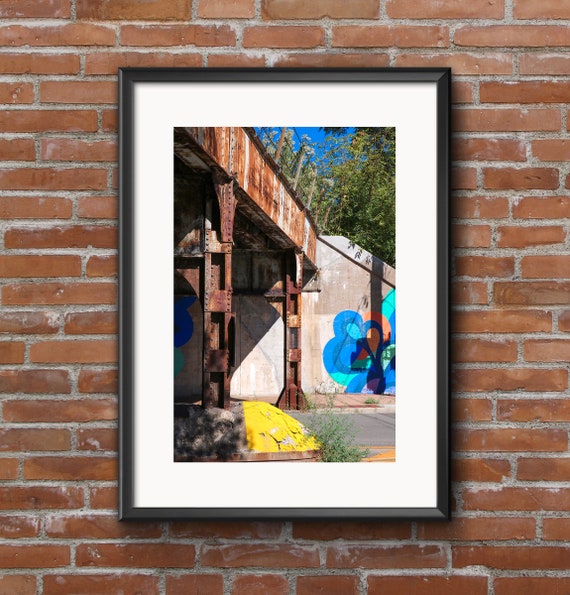This is a detailed photograph showcased within a carefully framed display on a red brick wall, interspersed with white or gray mortar. The photograph is bordered by a sleek black frame, accompanied by a white mat board that emphasizes the central image. The central photograph captures an industrial scene featuring an old, rusty iron bridge supported by heavy metal legs. The bridge traverses the top portion of the image, connecting to a concrete structure prominently adorned with vibrant blue and orange graffiti artwork that adds a touch of creativity to the otherwise gritty setting. Below the bridge, there is a hint of a paved road or walkway, defined by a yellow curb or yellow-painted bricks. Trees can be seen in the background, suggesting that this moment was captured on a bright, sunny day. The detailed and evocative scene is a testament to urban decay meeting artistic expression.